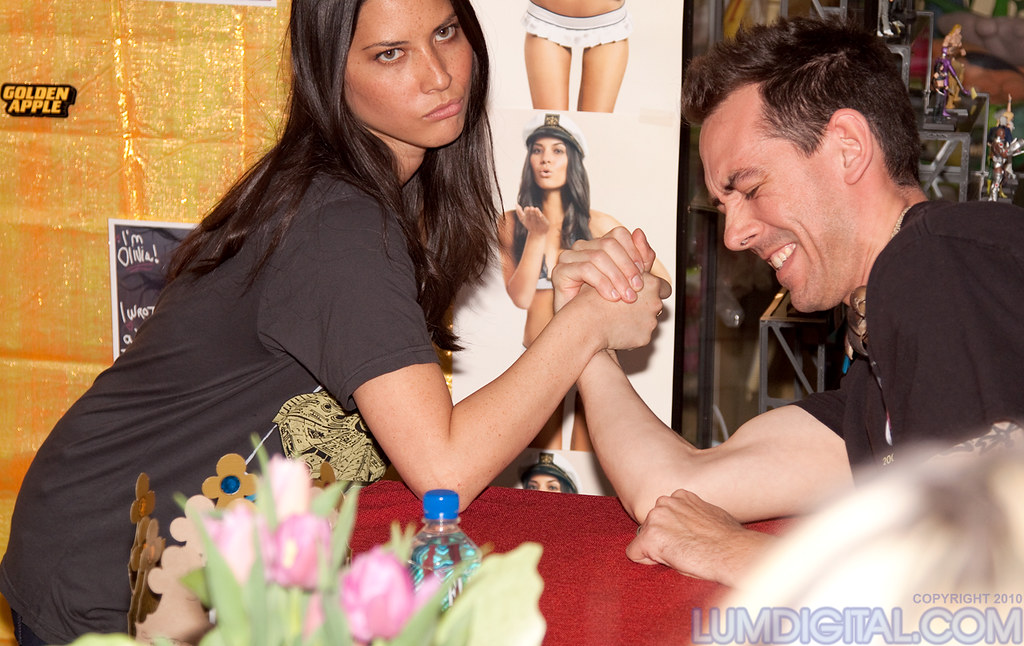The photograph showcases a dynamic arm-wrestling scene between a woman and a man, both dressed in black short-sleeved t-shirts. They are positioned slightly off-center, with the woman on the left and the man on the right. The woman, who has a stern expression, appears to be in a strong position, suggesting she might be winning, while the man is mugging comically as if he is losing. Their elbows rest on a small table covered with a red tablecloth.

Behind them, the background is rich with various colors including red, white, blue, maroon, yellow, gold, orange, gray, and brown. Adorning the wall are pictures of the woman dressed in lingerie and a captain sailor hat, indicating a potentially promotional or thematic setting. In the immediate foreground, there is a slightly out-of-focus bouquet of pale pink and green flowers. Additionally, a transparent water bottle with a blue cap is visible near the table.

The image exudes a professional vibe, possibly captured during a specific event by Loom Digital, as noted by the "Golden Apple © 2010 Loom Digital.com" text visible. The man also wears a lanyard, adding to the promotional feel.